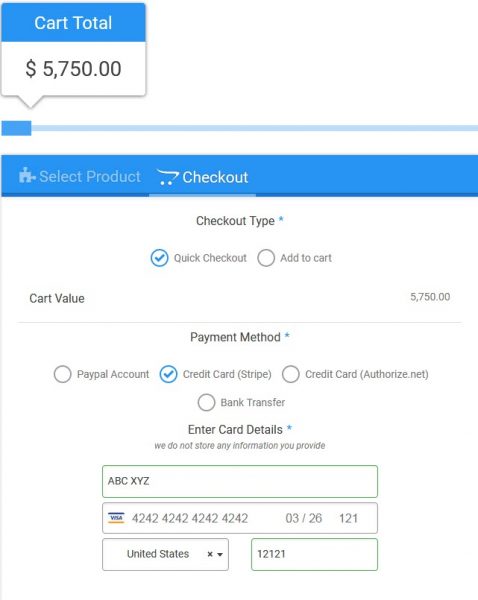The image depicts a detailed checkout page for an online shopping cart with a total cart value of $5,750. The page features several selectable options including 'Checkout,' 'Quick Checkout,' and 'Add to Cart.' Users can choose from various payment methods: PayPal, credit card via Stripe and Authorize.net, and bank transfer. In this instance, the credit card option has been selected, prompting the user to enter their card details. A note assures that no information provided will be stored. Four fields are visible, likely for card information, expiry dates, country, and additional relevant details. The overall color scheme includes white with black text, complemented by blue accents against the white background.